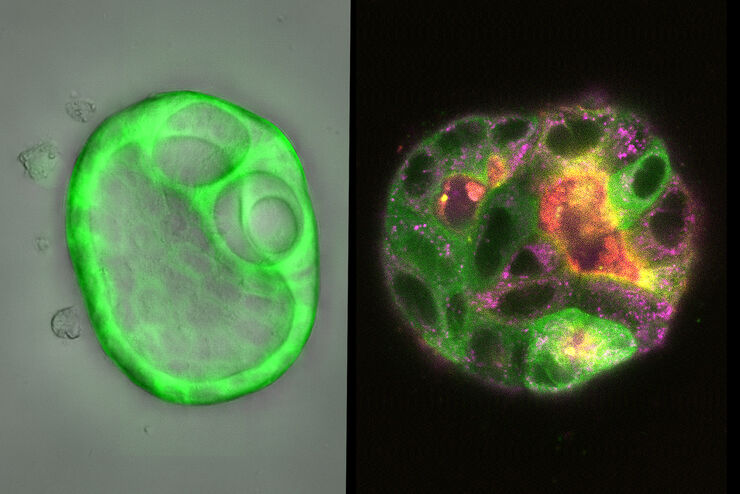This caption describes two side-by-side images showcasing what appears to be a microscopic view of a green, gel-like organism or molecule. 

On the left side, set against a whitish-gray background, there's a neon green, oval-shaped blob. This blob is semi-transparent in the center but has thick, bright green, and opaque edges that appear somewhat smooshy. Within this green oval, there are two additional smaller green circles positioned at the top right. These circles share the same smooshy texture and transparency in their centers, with a smaller hole visible beneath them.

The right side contrasts sharply with a dark black background and features a colorful, greenish-purple circular blob. This green blob has an array of vibrant hues including purples, reds, yellows, and light purples, almost like gems encrusted within it. It displays various specks and holes in shades of green and darker greens, with additional splotches of orange bordered in yellow. Together, these images highlight the diverse textures, colors, and forms of what looks like a gelatinous, molecular structure.